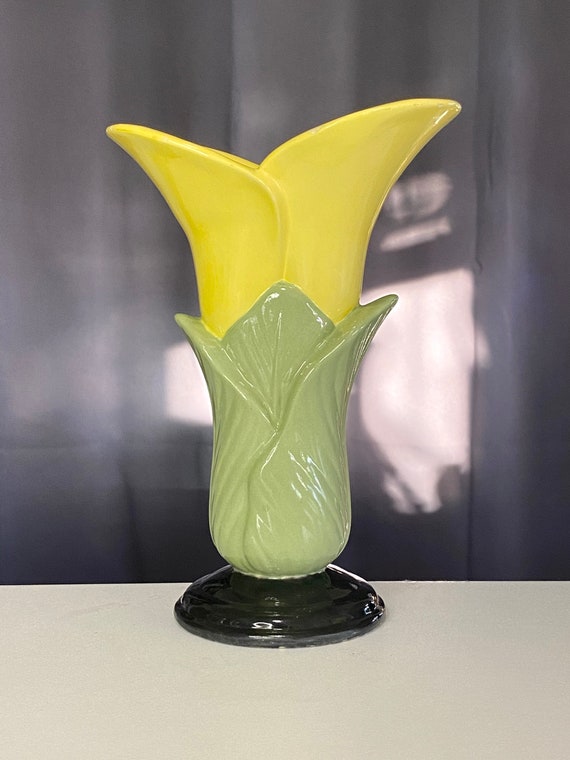The image is a color photograph, shot in portrait orientation, showcasing a striking piece of ceramic art shaped like a vase, which closely resembles a flower. The vase sits precariously near the edge of a white table, in a room with blue paneled walls. The shadow of a window, creating an intriguing light effect, is faintly visible in the blurred background. The vase itself features a black inverted saucer-shaped base, transitioning into a textured green leafy section that culminates in a yellow, lily-like petal opening at the top. The ceramic material boasts a shiny, glistening glaze, with the green leaves at the bottom having a distinctive rippled texture. The overall scene is devoid of any other elements, focusing solely on the vase, which stands empty. The background appears gray, with sunlight partially illuminating it.